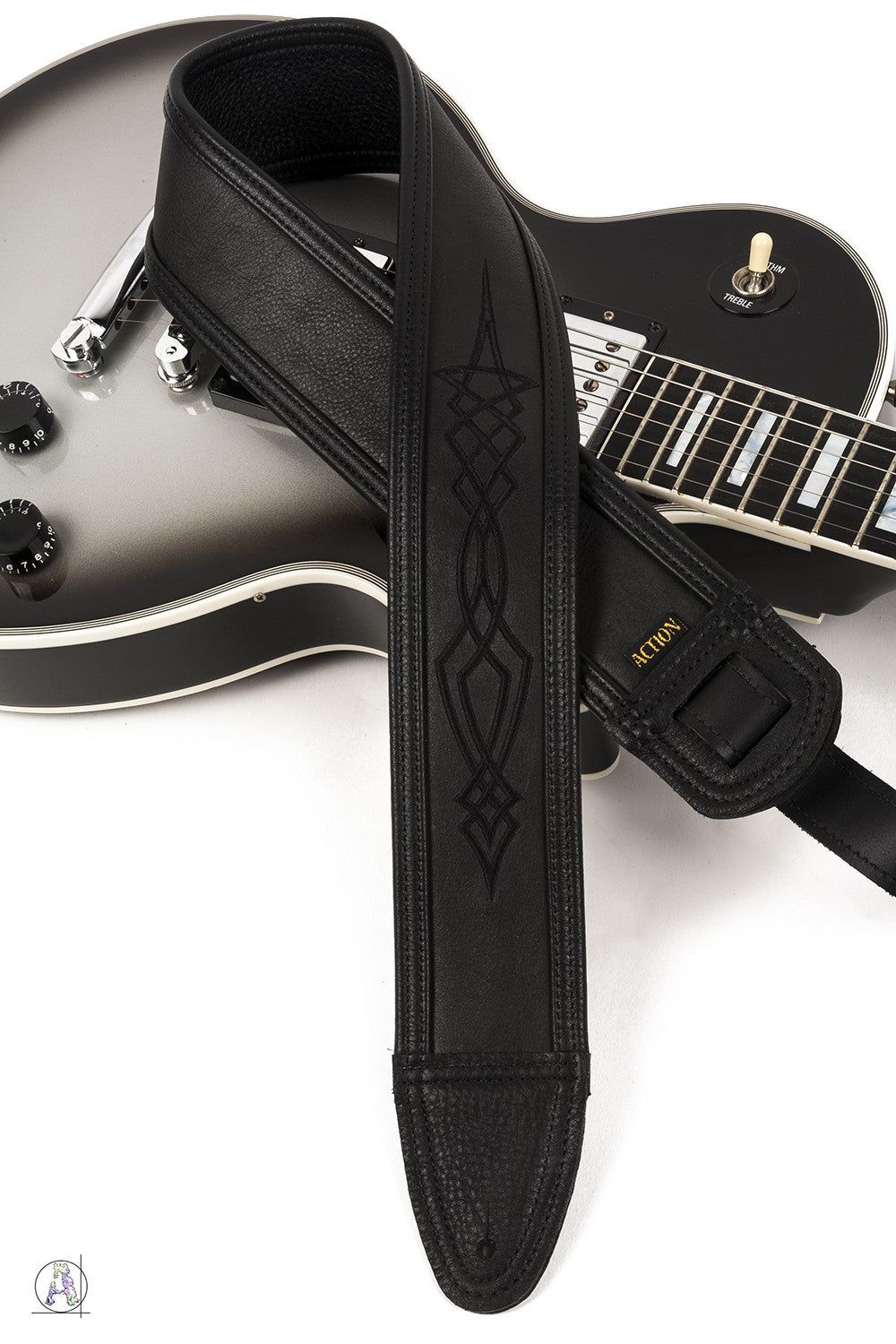In this image, we see a striking black and grey electric guitar, positioned on a clear white surface. The guitar, characterized by its shiny finish, features about seven strings, with shades of brown visible on the string area, creating a contrasting effect with the white strings themselves. It includes two dials and a switch located on the lower part of the body, adding to its detailed appearance. Draped over the guitar is a black leather or synthetic leather strap, which runs vertically across its surface. The strap is decorated with a Celtic-style design and prominently displays the word "ACTION" in blazing gold letters. The end of the strap is rounded, and overall, it exudes a vintage yet timeless charm, reminiscent of designs from the 90s.